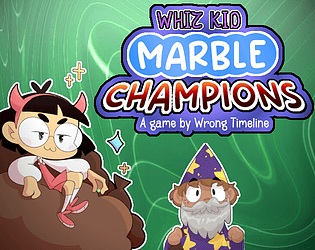The image appears to be a cover for a game titled "WizKid Marble Champions" by Wrong Timeline. The green background, reminiscent of grass, is adorned with white marbling and lines. Prominently, the text "WizKid" is in a blend of purple and pink, "Marble" in white on a blue background, and "Champions" in red with a white outline on a purple background. The central figures are two cartoon characters. On the left, a small wizard in a purple gown and cap, both decorated with yellow stars, sports a white beard and mustache. To his right, a little girl with black hair, red devil horns, and large eyeglasses is wearing a pink dress with white sleeves, white socks, and pink shoes. She appears to be sitting on bags of some kind, possibly suggesting wealth or rewards in the game. Both characters are facing the viewer, adding a sense of engagement to the image.